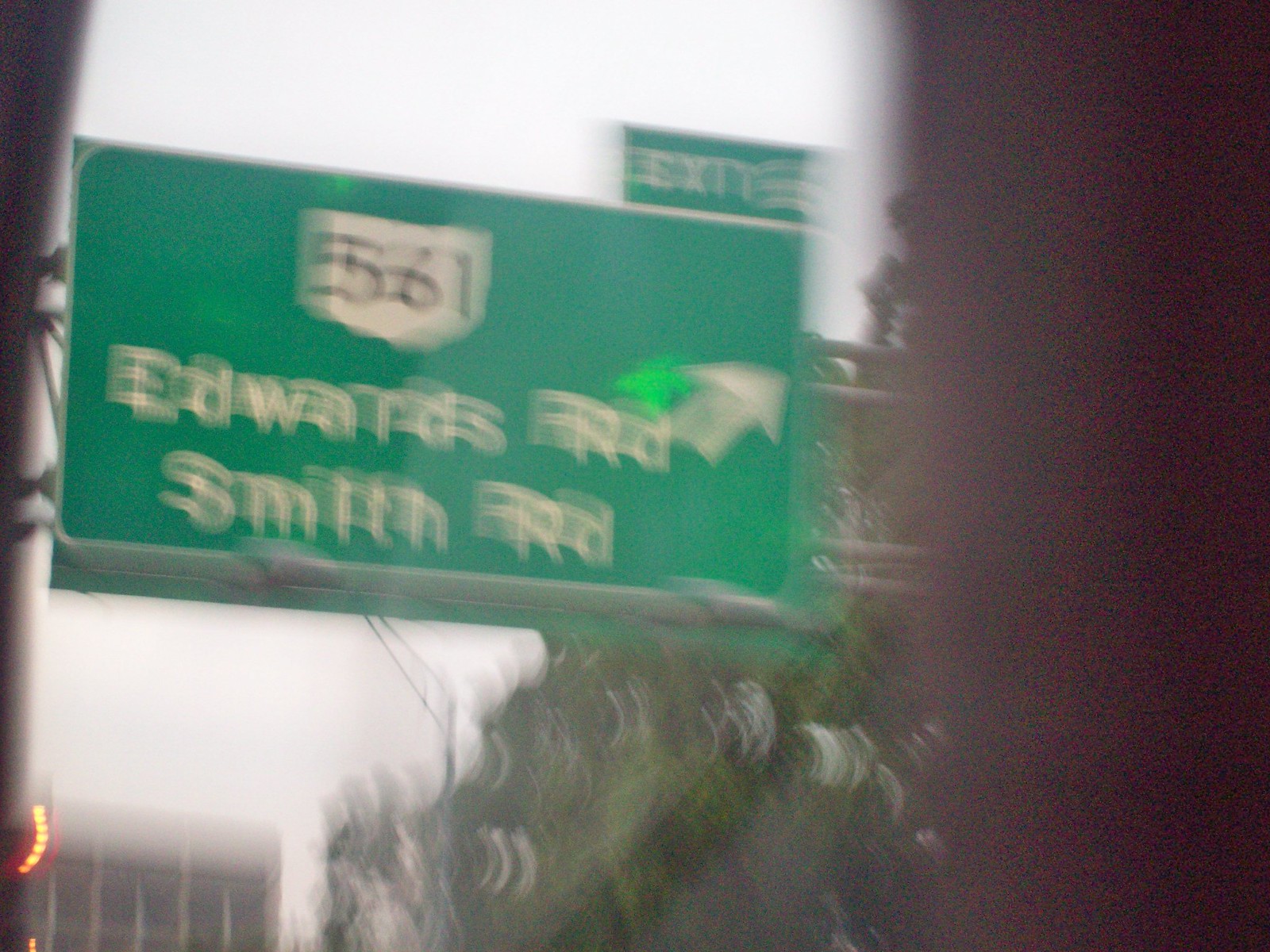In this image, there is a very blurry road sign prominently displayed. A dimly lit sky forms the backdrop, interspersed with patches of darkness, which partially obscure what appears to be a fence and a tree. The main sign, mounted on a light pole, consists of two distinct green sections. The smaller section at the top likely indicates "Exit 56" in white lettering on a green background. Below this, a larger green sign bears a white box with "561" inscribed in black numbers. This larger section also features directional guidance, pointing to "Edwards Road" and "Smith Road," with an arrow directing to the right.